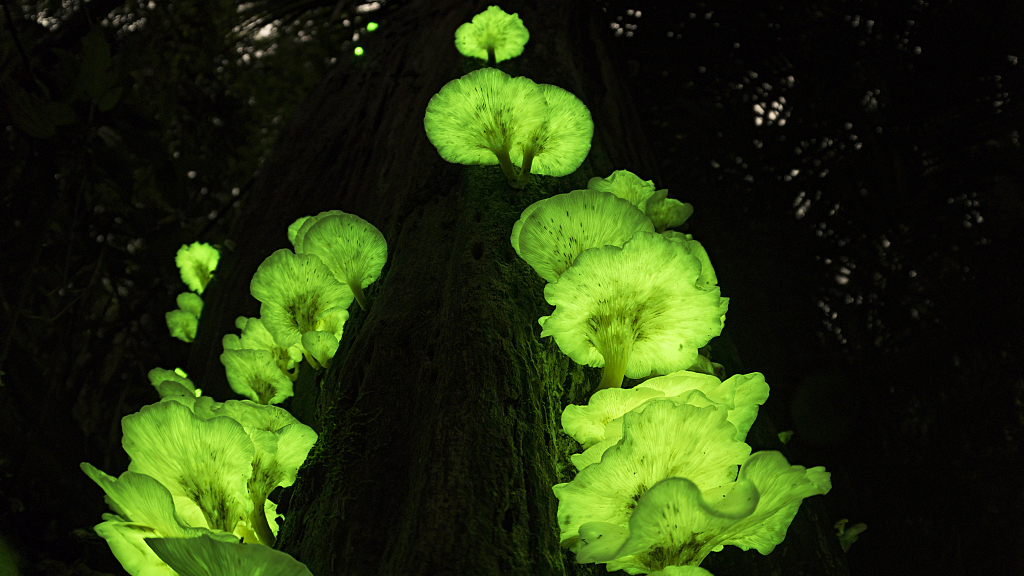The image is a horizontally rectangular outdoor photograph depicting a dark, dense forest with very faint hints of sky visible through a thick canopy. At the center of the image stands a large tree trunk, its rough bark dimly outlined by the surrounding darkness. Growing from this tree trunk are large, bioluminescent fungi, resembling big, glowing green mushrooms. These mushrooms have thin cylindrical stems and wide, flat caps that emit a bright, luminescent green light. They form multiple rows traveling upwards on both sides of the tree, with the ones on the left starting large at the bottom and gradually becoming smaller as they ascend. The overall scene has a mystical, almost ethereal quality, dominated by the vibrant green glow of the mushrooms against the otherwise shadowy forest backdrop.